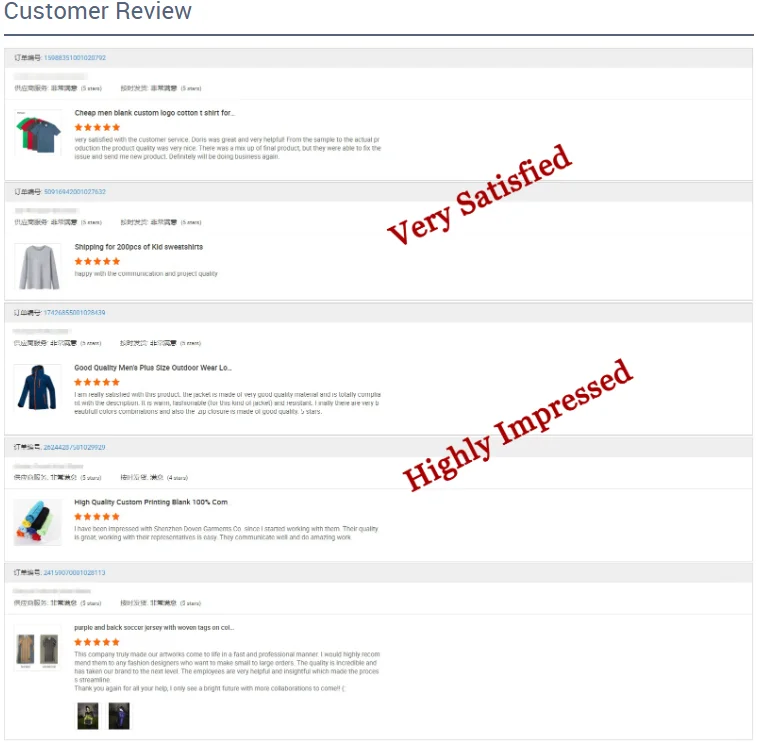**Detailed Caption:**

A screenshot from a desktop computer featured on a review site. The header reads "Customer Review," showcasing five separate product reviews. The layout, with its wide dimensions, indicates it's not captured from a mobile or tablet device. Each review is visually annotated in bright red text, with the first two reviews marked as "Very Satisfied" and the subsequent two labeled "Highly Impressed." 

The first review is for "cheap men's blank custom logo cotton t-shirts," awarded a five-star rating. The detailed feedback highlights:
- Exceptional customer service, notably praising Doris for her assistance.
- High-quality product from sample to final production.
- A minor mix-up in the final product, which was efficiently resolved, prompting the reviewer to express a strong likelihood of future business.

Non-Latin characters appear mixed in the site’s interface, but all review content is in English, suggesting a possible international platform, perhaps a B2B site. The fifth review, while present, lacks any additional annotation in red text.